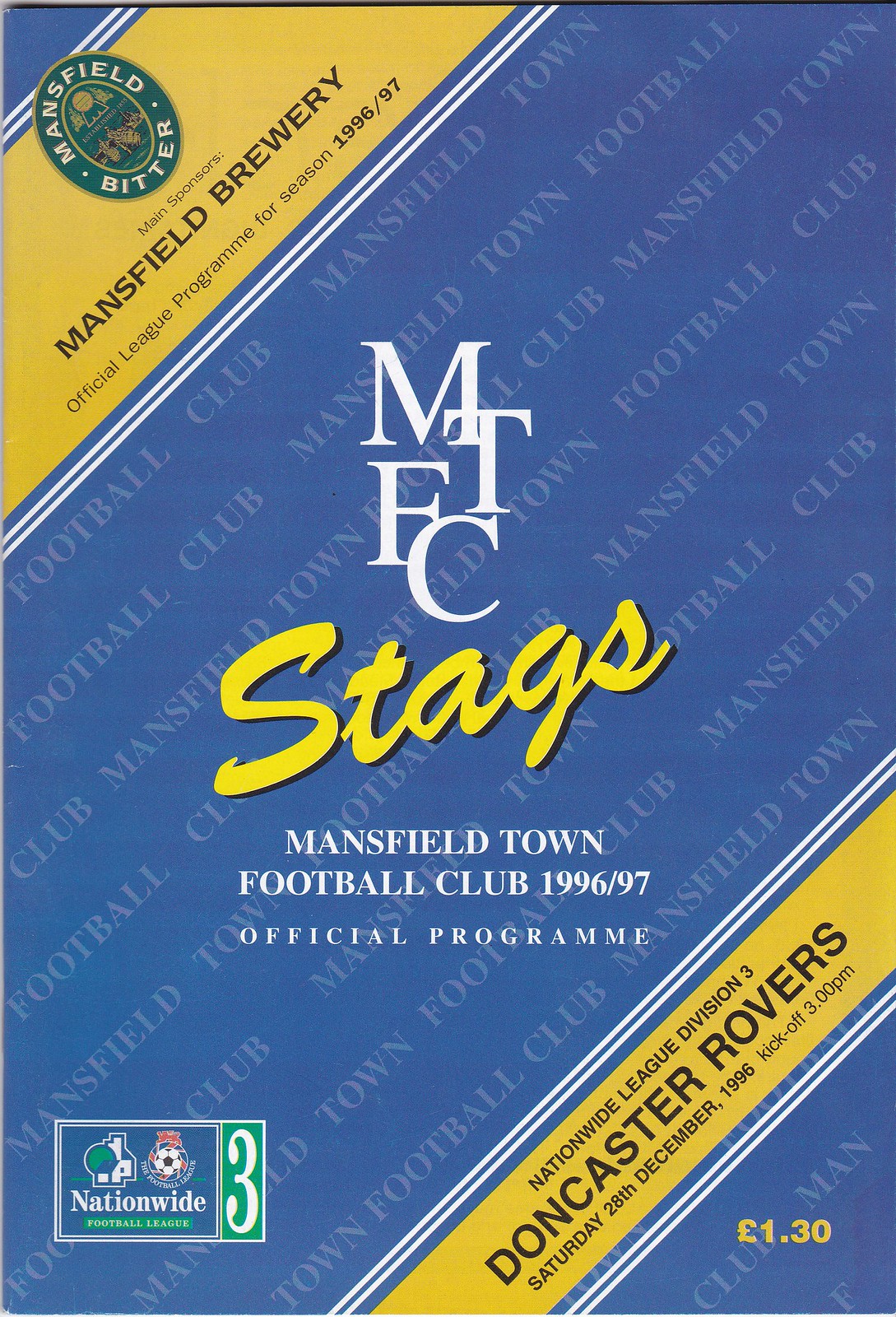The image depicts the cover of the 1996-97 official program for Mansfield Town Football Club, primarily designed in a blue background with the text "Mansfield Town Football Club" repetitively running diagonally across. The title "Stags" is prominently displayed at the center in an elegant cursive font, accompanied by the letters "MTFC" in a bold, stylized logo above it. The poster features two oblique yellow stripes: one near the upper left corner and the other near the lower right corner. The top left stripe includes an oval emblem stating "Mansfield Bitter," and below it reads "Mansfield Brewery official league program for season 1996-97," indicating their sponsorship. The lower right stripe includes details about a specific fixture, mentioning "Nationwide League Division 3 Doncaster Rovers," along with the date, time, and price of the program (£1.30).